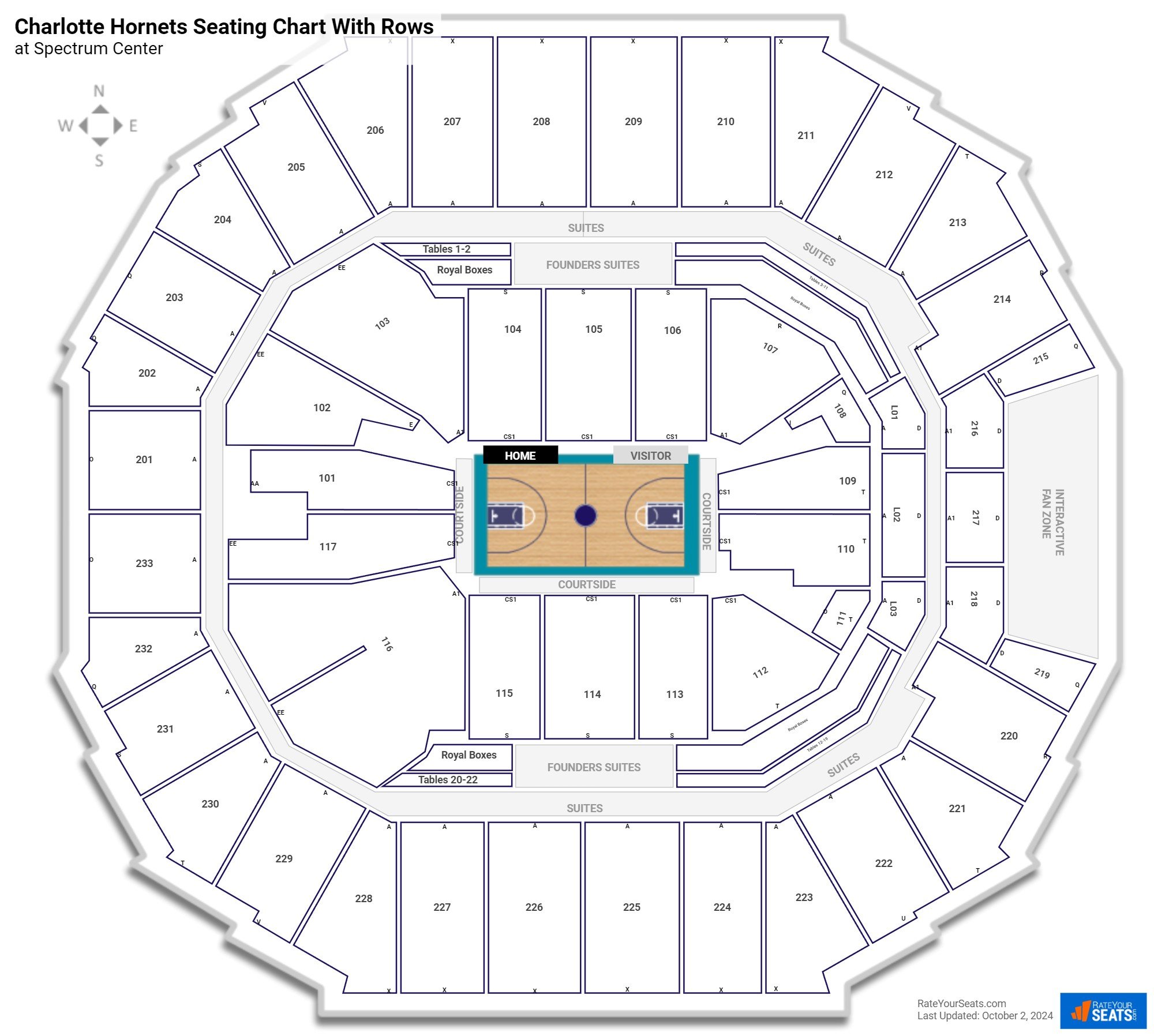This image depicts a detailed blueprint of a stadium, specifically the Spectrum Center, with a seating chart for the Charlotte Hornets prominently featured. In the top left corner of the blueprint, "Charlotte Hornets Seating Chart" is displayed in bold black letters, with "Spectrum Center" written directly below in smaller, non-bold text. A compass rose is positioned underneath, indicating the cardinal directions—north, east, south, and west—with a triangle pointing towards each direction. 

To the right of the compass, the blueprint showcases the stadium's seating arrangement. Due to the image's small and blurry sections, it’s challenging to discern all details clearly, but each seat's section is marked with a number. The sections are varied in size and shape, creating an intricate and diverse seating layout.

At the center of the stadium, the basketball court is depicted with precise detail. A dark blue circle is situated at the middle of the court, intersected by a vertical line. The court is bordered in teal on all four sides, and the interior court area is shaded in a light brown color. Additionally, a black rectangle in the top left corner of the court area is labeled "Home," and a gray rectangle on the top right side features another, less discernible designation.